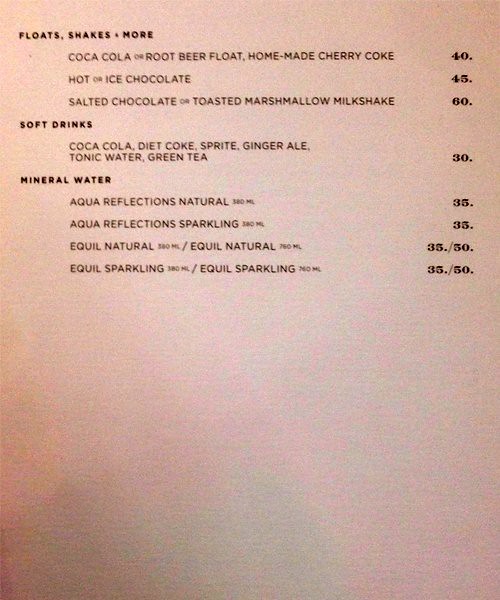The menu, presented on a vertical, rectangular piece of pinkish-hued paper, is simply laid out in black text with light illuminating certain areas. The top half is dedicated to three sections: "Floats, Shakes, and More," "Soft Drinks," and "Mineral Water."

1. **Floats, Shakes, and More:**
    - **Coca-Cola or Root Beer Float**
    - **Homemade Cherry Coke** - 40 cents
    - **Hot or Iced Chocolate** - 45 cents
    - **Salted Chocolate or Toasted Marshmallow Milkshake** - 60 cents

2. **Soft Drinks:**
    - **Coca-Cola, Diet Coke, Sprite, Ginger Ale, Tonic Water, Green Tea** - 30 cents each

3. **Mineral Water:**
    - **Aqua Reflections Natural (380 ml)** - 35 cents
    - **Aqua Reflections Sparkling (380 ml)** - 35 cents
    - **Equil Natural (380 ml)** - 35 cents
    - **Equil Natural (760 ml)** - 50 cents
    - **Equil Sparkling (380 ml)** - 35 cents
    - **Equil Sparkling (760 ml)** - 50 cents

The bottom half of the page remains blank, emphasizing that the menu content only occupies the top portion.